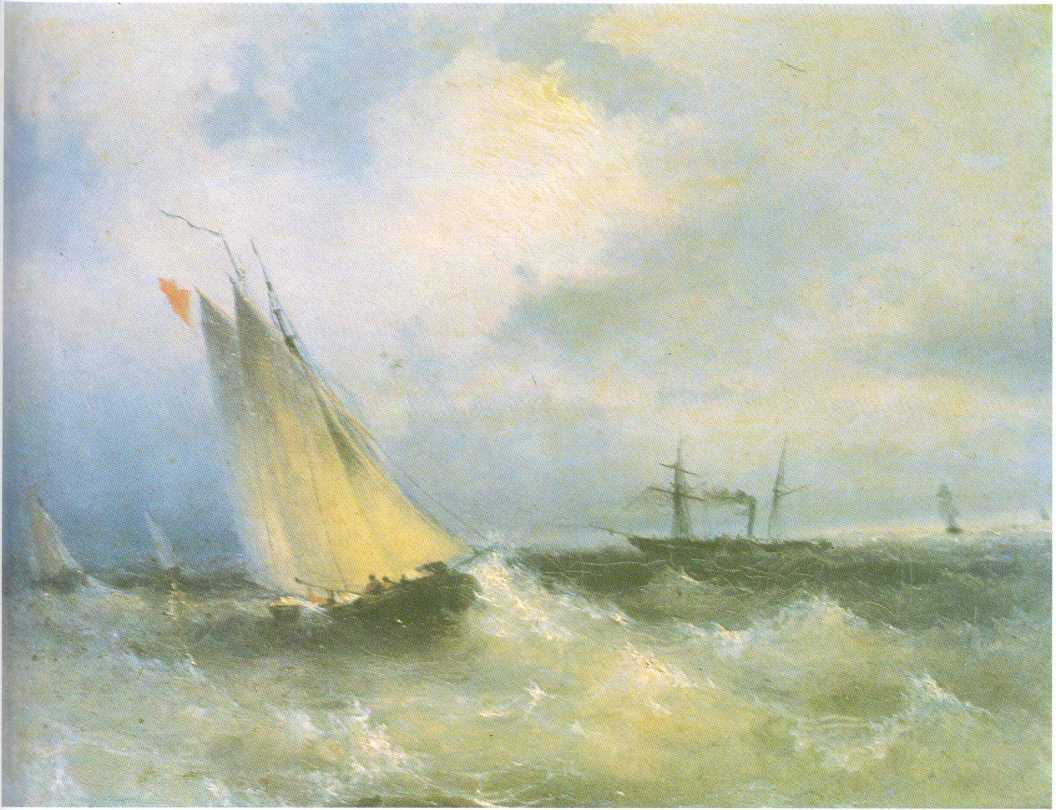This is a richly detailed watercolor painting depicting a tumultuous sea scene. The sky is painted in hues of light baby blue but appears stormy and overcast, filled with dark gray, fluffy clouds. The choppy waters below are a blend of white, yellow, olive green, and murky shades, suggesting rough and tumultuous waves. In the foreground, a sailboat is prominently tilted to the left, battling the fierce waves. The boat features an orange and red flag fluttering behind the rear mast, indicating it is moving from left to right due to the wind. Although the figures on the boat are merely specks of color, they can be seen attempting to steady the vessel. Behind this sailboat, there are at least three other boats, including a larger twin-masted schooner possibly steam-powered, identifiable by the smoke stack emitting smoke. The overall scene is portrayed with an array of neutral colors, providing depth and detail while maintaining an impressionistic and less realistic style. This evocative painting captures the raw energy of the sea, the determination of sailors, and the brooding atmosphere of a stormy seascape.